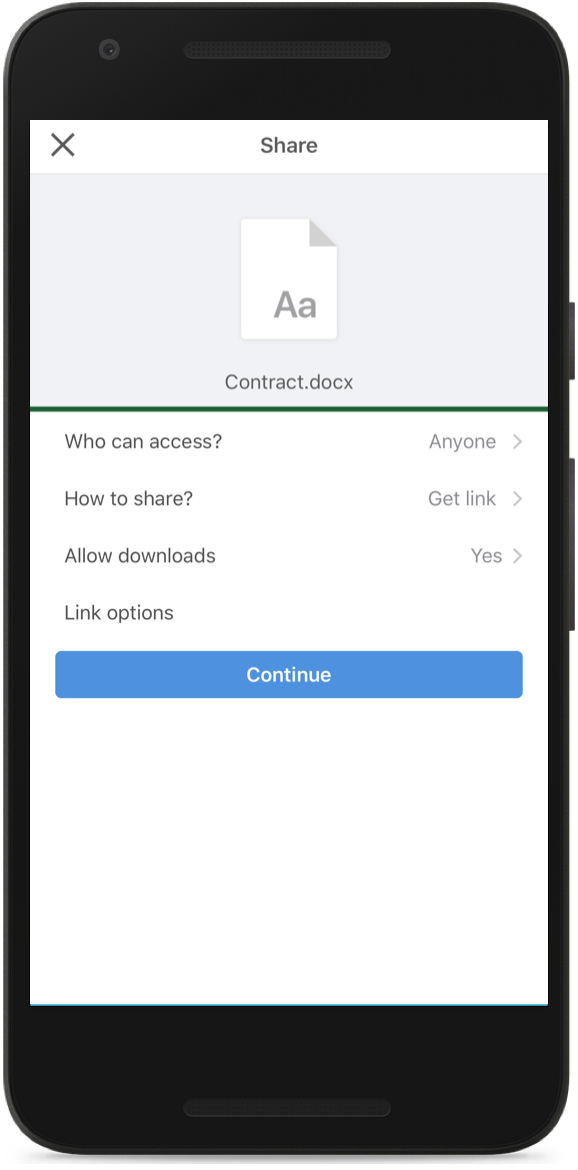A black smartphone displays a white screen showcasing a website. At the top center of the screen, the word "Share" is prominently displayed, accompanied by an "X" icon in the top left corner. Below these, there's a light gray text box featuring a paper symbol with a folded upper right corner, alongside a capital "A" and lowercase "a."

Directly beneath this icon, the text "contract.docx" appears, underlined by a vivid green line. On the left, the phrase "Who can access" is written, and to the right, "Anyone" is followed by a right-facing arrow. Below that, the options "How to share and get link," "Allow downloads - Yes," and "Link option" are listed sequentially, each accompanied by a right-facing arrow, except for the last option.

At the bottom of the screen is a blue button labeled "Continue" in white text. The rest of the screen is filled with blank white space. All textual elements range in color from light gray to black, ensuring clarity and readability on the display.